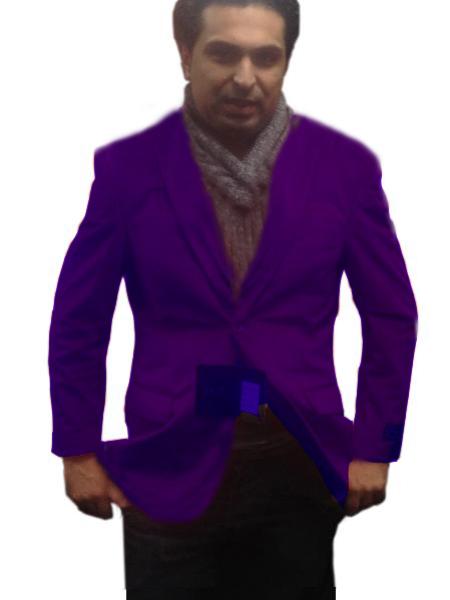The image portrays a middle-aged man of medium skin tone, likely of either Middle Eastern, Asian, or Asian-Indian descent, captured from mid-thigh up to just above his hairline. He is facing the camera directly, his expression neutral with his mouth slightly open as if he has just spoken. His hair is black, possibly dark brown, and he appears to be in his mid-40s with a slightly balding hairline. He is dressed in a striking dark purple jacket that catches the eye, under which he wears a medium gray jumper and a thin gray scarf wrapped around his neck. His attire is complemented by black pants that are partially visible, ending just below the groin where the image cuts off. His hands are in his jacket pockets, with a noticeable blue square object slightly protruding from under the jacket's button, adding an additional point of interest. The man extends the sides of his jacket with each hand, suggesting he might be showcasing it, although his demeanor does not strongly suggest a modeling pose. The background is plain, ensuring all focus remains on the gentleman's distinct appearance.